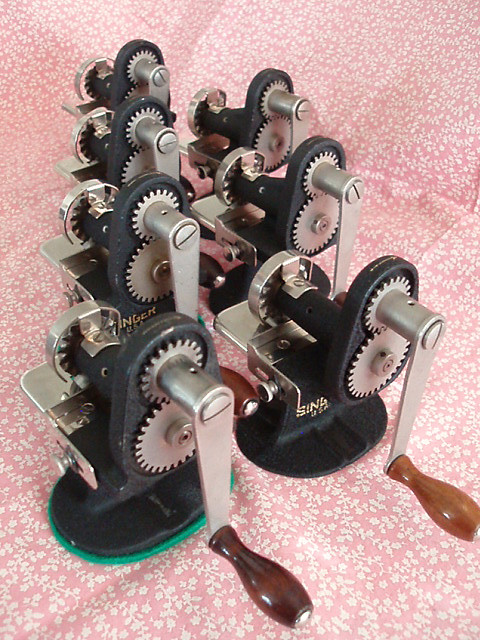In the image, a decorative hot pink fabric with small white floral designs serves as the background. The fabric appears to have been previously folded, evident from the visible creases, especially in the upper right-hand corner. Atop this fabric, there are seven old-school pencil sharpeners, aligned in two diagonal rows—four in the front row and three in the back. Each sharpener consists of exposed inner mechanisms, including interlocking metal gears and a crank handle. The handles are metallic and fitted with small brown wooden grips. These mechanisms are partially encased in black plastic bases. Two of the sharpeners display the branding "Singer USA." The overall composition combines the intricate mechanical details of the sharpeners with the vibrant, floral textile background, creating a visually intriguing contrast.